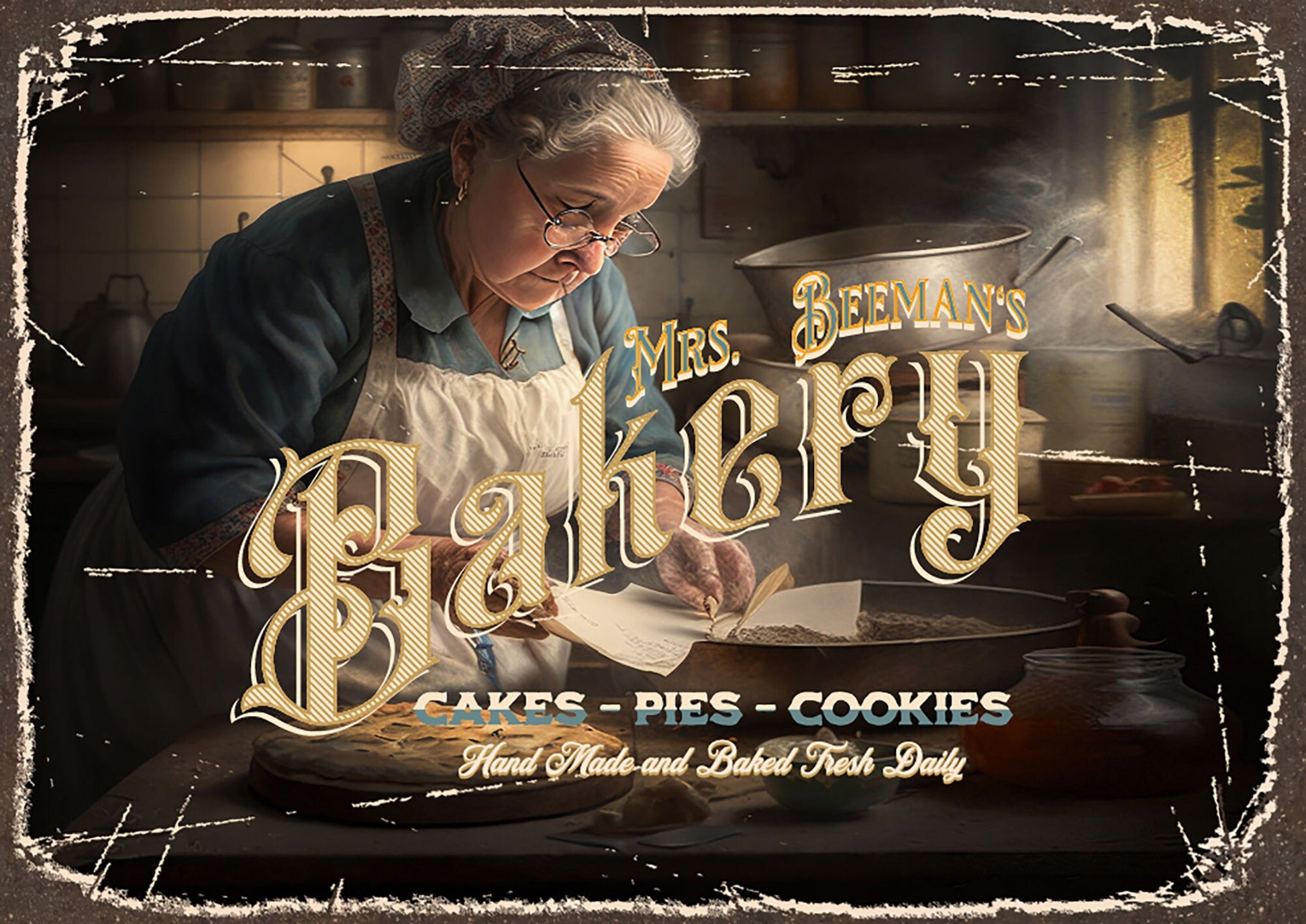The photo appears to be a timeworn, slightly bent image with a faded gray border, adding a touch of nostalgia. The sign reads "Mrs. Beeman's Bakery" in charming, striped green and yellow letters. Below, in pristine white lettering, it advertises the bakery's offerings: "Cakes, Pies, and Cookies, Handmade and Baked Fresh Daily." At the center of the scene is an elderly lady with gray hair and glasses, dressed in a blue dress and a white apron. She intently examines her recipes, with a large pan before her and a substantial pot on the stove in the background, epitomizing her dedication and bustling activity within the bakehouse. The image captures the essence of a bygone era and the warm, industrious spirit of Mrs. Beeman as she bakes her delightful treats.